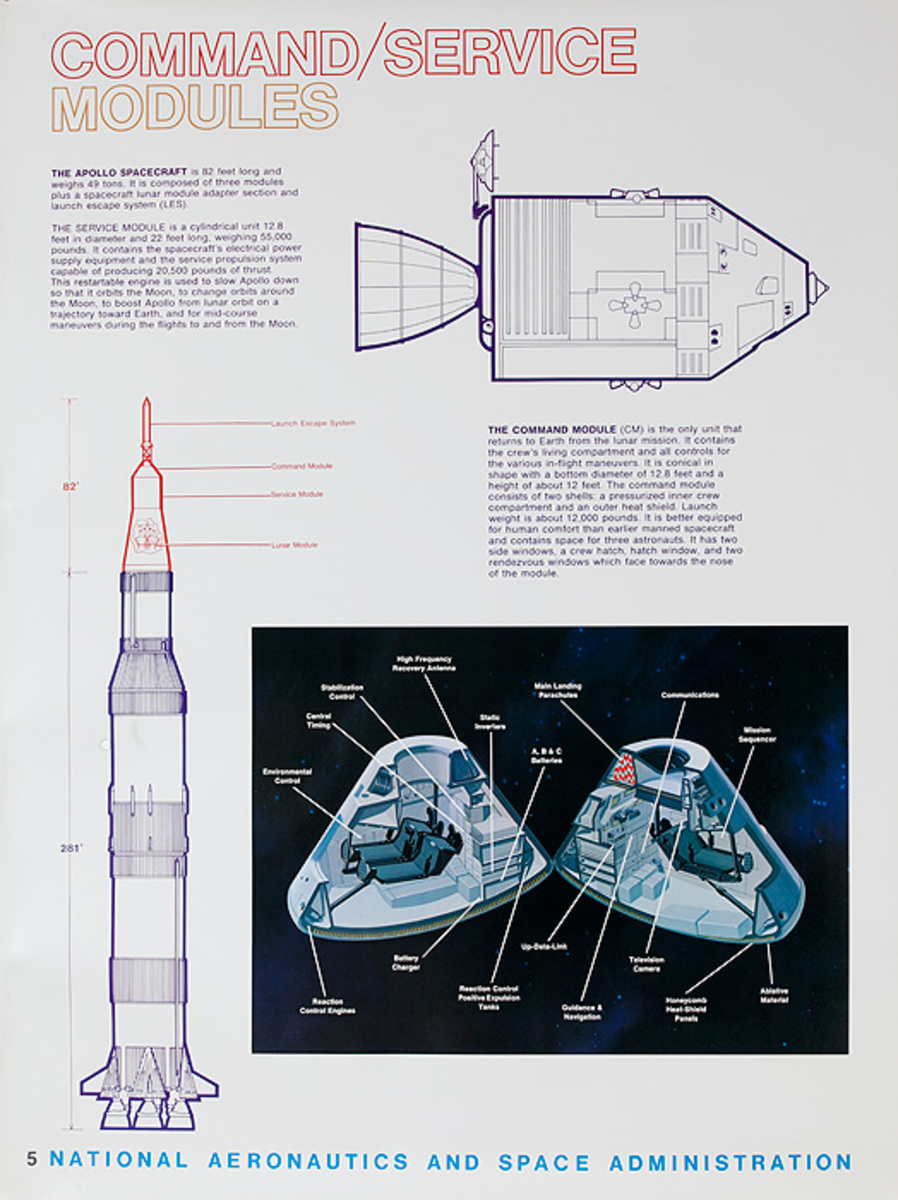The image is a vertical rectangle with a gray background, resembling a page from a book or a sign, most likely digitally created due to the clarity of the text and images. At the top, "Command/Service" is written in transparent text with a red outline, and below it, "Modules" is in similar text with an orange outline. The number "5" stands out in bold black at the bottom, beside the bold blue text "National Aeronautics and Space Administration."

The image is split into three sections, with detailed captions and diagrams. The top left section features a paragraph in bold purple text titled "The Apollo Spacecraft," elaborating on the overall design and function of the spacecraft. To the right of this text, a detailed drawing or schematic of the Apollo spacecraft provides insight into its structure. This is labeled "The Command Module" in bold letters, with further explanatory text below it.

On the left side, there's another striking visual of a rocket ship in purple with a red tip, accompanied by a measuring scale, highlighting the dimensions—82 inches in red and 251 inches in navy blue. The bottom right section contains an image with a black background, displaying parts of the spacecraft with white text explaining various features, though the text is too small to read from the overview.

Overall, the image serves as an informative guide to the components and structure of the Apollo command/service module, complete with detailed diagrams and descriptive text.